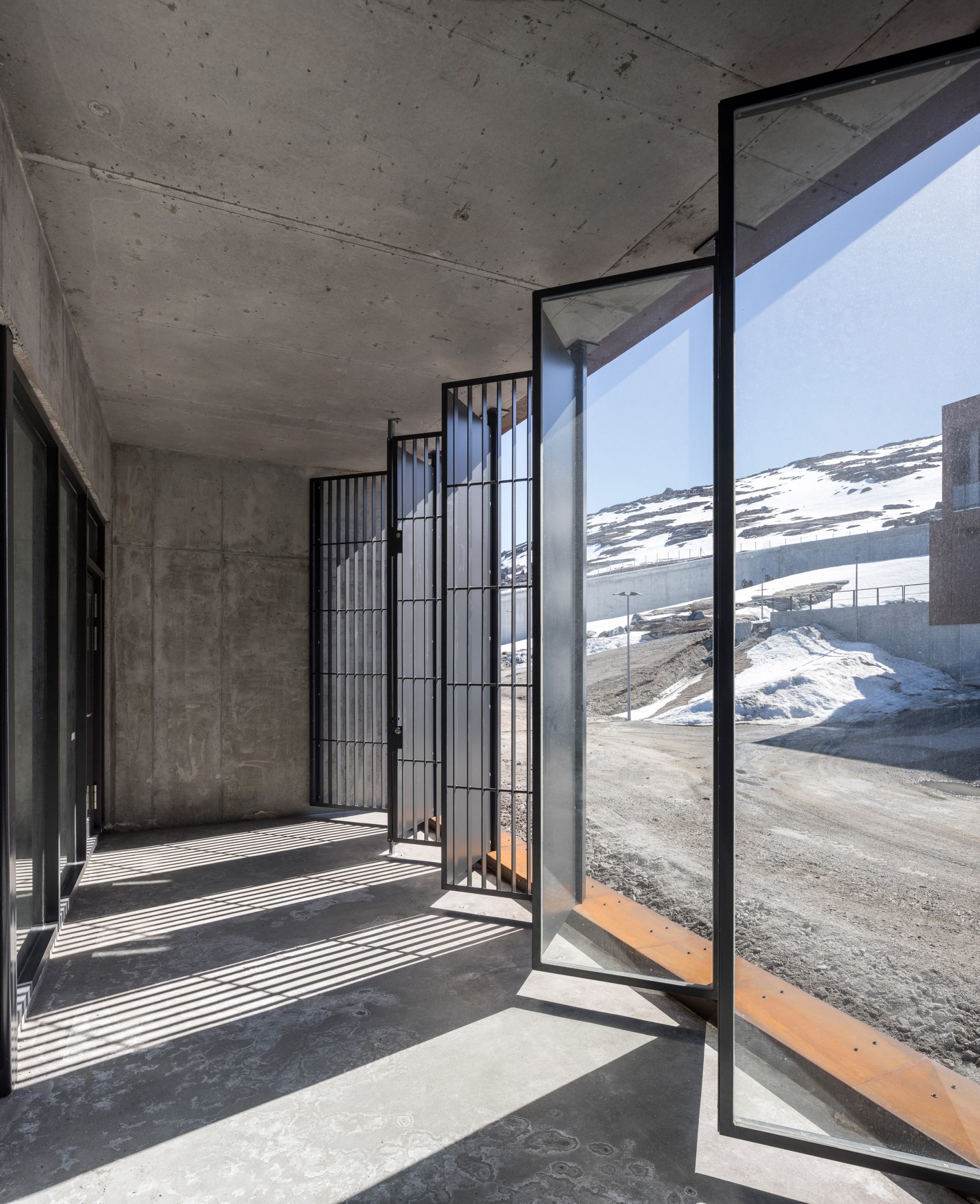The image depicts an interior view of a concrete building that appears to be situated in a cold, snowy environment, likely indicating heavy snowfall outside. The scene is dominated by a spacious hallway or breezeway lined with black-framed glass sliding doors and large windows. Some of the windows, especially towards the back, are covered with metal bars, casting a distinct barred light pattern onto the concrete floor, suggestive of a jail or an industrial facility. The exterior view, visible through the clear glass windows, reveals a dirt road leading to a large, barren hill with patches of scattered snow, emphasizing the desolate and cold atmosphere. An adjacent brick building and a fence are partially visible in the background, enhancing the isolated feel of the location. Additionally, the interplay of light through the variously framed windows creates visually interesting patterns reminiscent of geometric shapes like a Toblerone. Overall, the stark contrast between the bare, concrete interior and the sparse, snow-covered exterior reinforces the impression of a cold and possibly institutional setting.